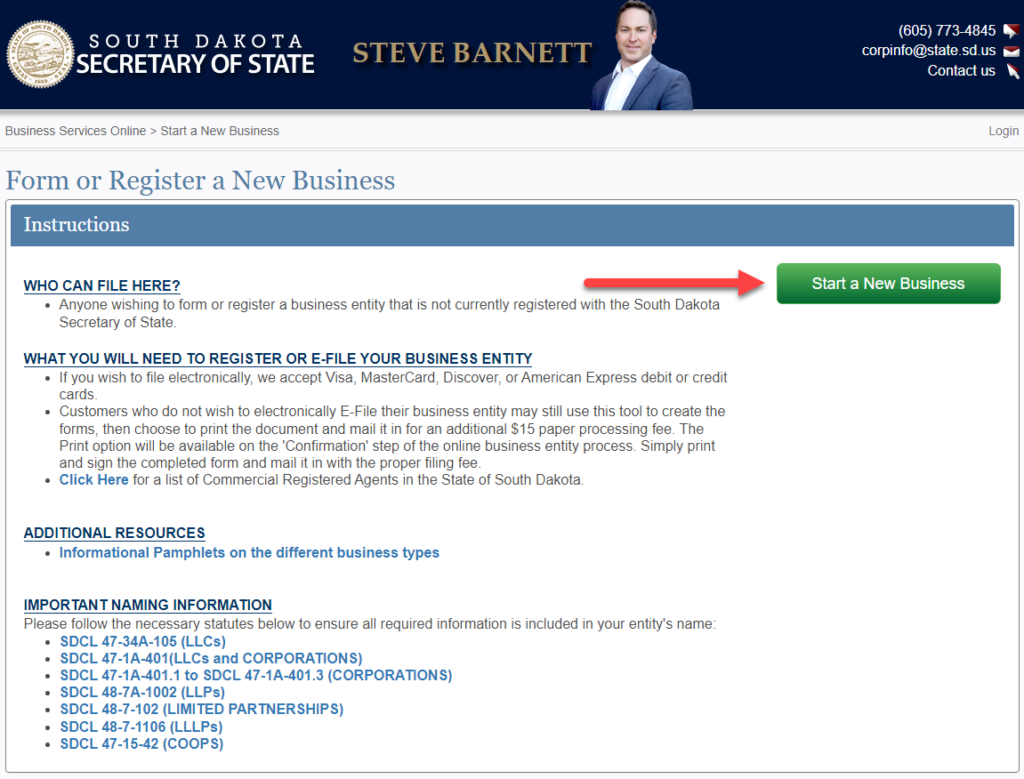A screen capture from a computer monitor displaying the South Dakota Secretary of State website. At the top of the page, a black banner features the grey state logo on the left, with "South Dakota Secretary of State" written in grey and white lettering. Prominently centered in yellow lettering is the name "Steve Barnett." On the right side of the banner, there is a photograph of a man appearing to be in his early 40s, dressed in a suit and dress shirt but without a tie. In the upper right-hand corner, contact information is provided, including a phone number, an email address, and a "Contact Us" link.

Below the banner, the page background is predominantly white with the header text stating "Form or Register a New Business." At the top of this section, a large grey-outlined text area features a blue bar labeled "Instructions" in white text. Running down the left-hand side of the page, a list of categories is displayed: "Who Can File Here," "What You'll Need to Register or E-File," "Your Business Entity," "Additional Resources," and "Important Naming Information."

On the top right corner of this main white section, beneath the blue instruction bar, a prominent green rectangular button with "Start a New Business" written in white letters is displayed. To the left of this button, a bold red arrow points directly at the green "Start a New Business" box, emphasizing its importance and location.